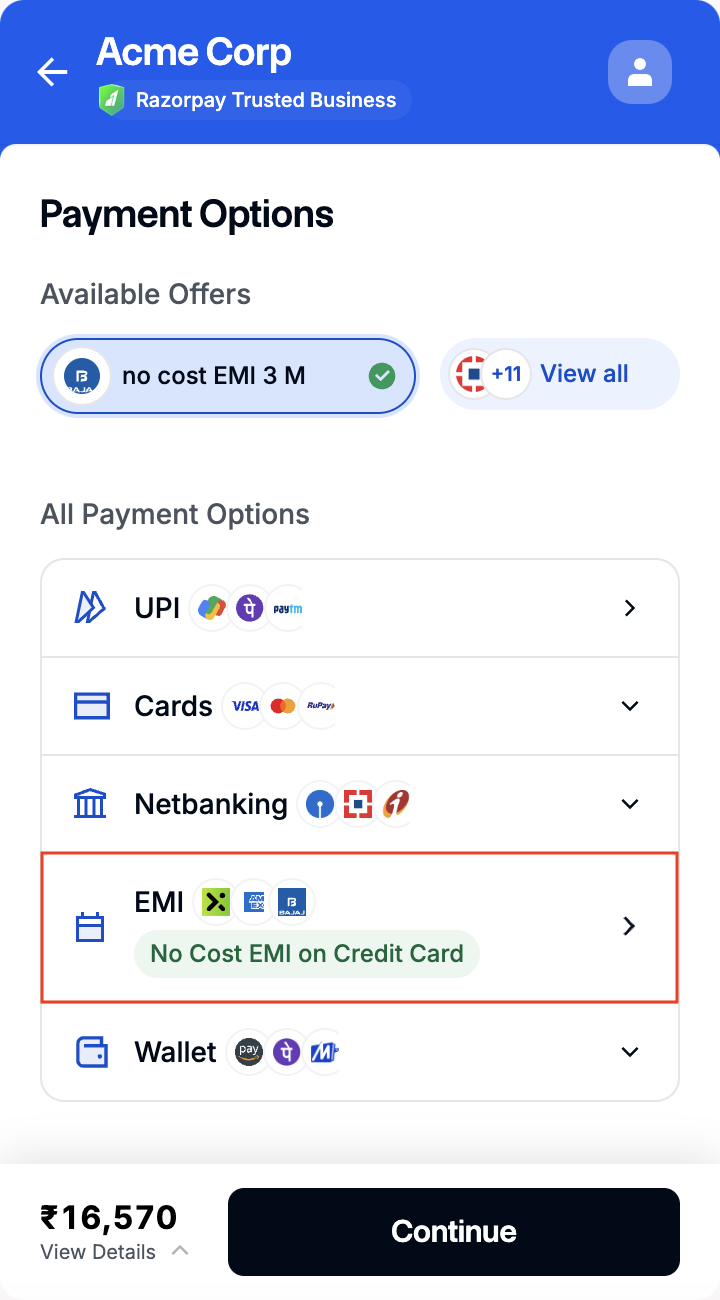This image is a cropped screenshot of a checkout page from Acme Corp. At the top, there is a blue header featuring a square icon with the letter "A" and the text "Acme Corp" in bold white letters beside it. Below the header is a semi-transparent white banner displaying a green logo with a white checkmark, alongside the words "Razorpay Trusted Business" in white. On the right of the banner, a dropdown box allows users to change the font size.

The body of the page is predominantly white. At the top left, the text "Cards, UPI, and More" appears in bold black font. Below, there is a vertical list of accepted payment options starting with "Card" and featuring circular logos for Visa, MasterCard, and American Express, with an ellipsis indicating additional options. The next option, "UPI/QR," similarly displays circular logos below with an ellipsis for more choices. 

Next, the "Net Banking" option is listed in bold gray font with "All Indian Banks" underneath. Following that is the "Wallet" option, showing icons for PhonePe and others. The final option is "EMI," indicated in bold text with a green box on the right displaying "No Cost EMI Available." Below this, it states "EMI via Debit, Credit Cards, Axio, and More." A red box is edited around this section highlighting the "Click This" notice.